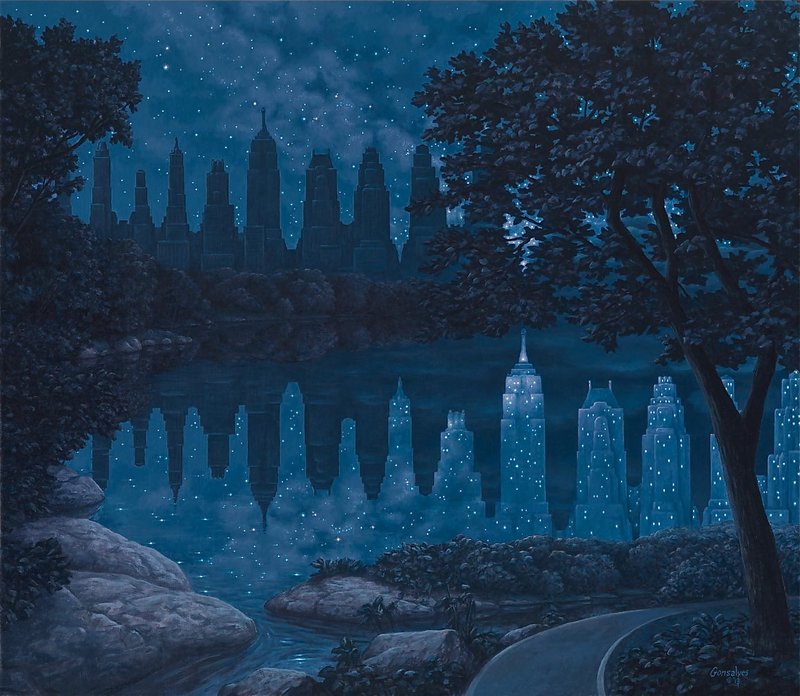This vibrant painting captures a serene nighttime scene transformed into an ethereal landscape. The starry sky at the top of the image casts a mystical light over the scene, dotted with twinkling stars. Towering skyscrapers with thin spires, though not fully illuminated, hint at a distant cityscape. In the foreground, large trees on both the left and right frame the image, their darkened branches adding depth and contrast.

A tranquil lake spans the middle of the painting, its reflective surface mirroring both the muted city skyline and the starlit heavens above. The reflections create an optical illusion: the illuminated buildings in the water appear as a continuation of the skyline, though they don bright lights unlike the actual structures. Intriguingly, the center of this reflection showcases a particularly luminous building that seems to be obscured in the real skyline by the trees, adding an element of mystery.

A winding road curves gently from the bottom corner, veering right past the tree on the edge. On the left side, the lake narrows into a small river that disappears into the distance. There’s an artful composition in the way the reflections blend into one another, merging into a single entity towards the bottom, creating a surreal quality. The dark buildings also blend indistinctly at the top, enhancing the dreamy and somewhat abstract nature of this nightscape painting.